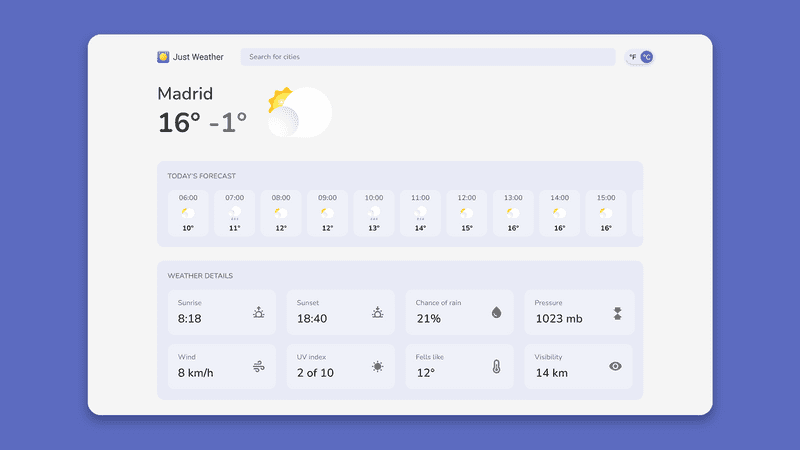A detailed weather forecast chart for Madrid, Spain, displays current and predicted weather conditions. The chart shows a sunny outlook with the temperature currently at 16°C, expected to drop to a low of -1°C. Throughout the day, temperatures will range from 10°C in the early morning, peaking at 16°C around 1 PM, and maintaining this high until approximately 3 PM.

Key weather details include:
- **Sunrise:** 8:18 AM
- **Sunset:** 6:40 PM (18:40)
- **Chance of Rain:** 21%
- **Barometric Pressure:** 1023 mbar
- **Wind Speed:** 8 km/h
- **UV Index:** 2 out of 10
- **Feels Like Temperature:** 12°C (although the actual temperature is 10°C)
- **Visibility:** Approximately 12 kilometers

The weather chart also features an option to search for different cities, with Madrid set as the default location.